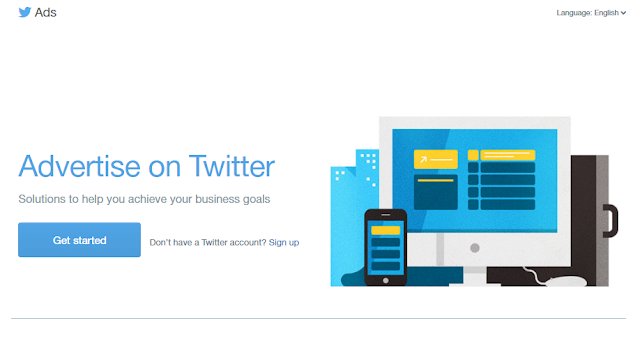In this image, set against a clean white background, we see a crisp screenshot from the Twitter advertising platform. Prominently located in the upper left corner is the iconic blue Twitter bird logo, immediately identifiable. Directly to the right of the logo, the word "Ads" is displayed in a subtle gray font. 

On the upper right corner, there is a small gray text indicating a pull-down button that reads "Language: English". Below this, on the left lower side of the image, in bold and large blue text, it states "Advertise on Twitter". Below this header, in smaller gray text, is the phrase "Solutions to help you achieve your business goals". 

Towards the bottom left, a noticeable blue action button is present with "Get Started" written in white text. Adjacent to this button, on the right side, there is an invitation for those who do not have a Twitter account, displayed in gray text: "Don't have a Twitter account?" Followed by a blue text link encouraging users to "Sign up".

On the right side of the image, there is an illustration depicting a black laptop, a modern black cell phone, and a sleek briefcase. In the background to the left, two towering high-rise buildings emerge, adding a professional and business-oriented context to the visual.